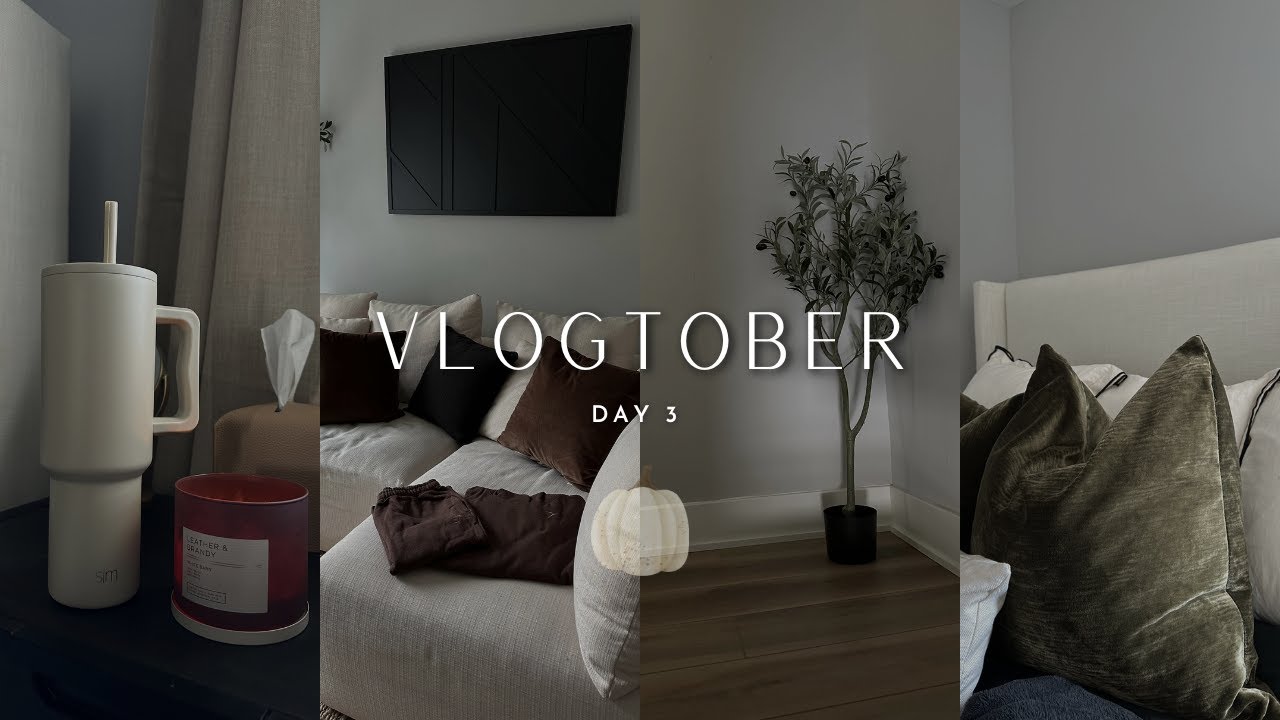Discover the epitome of cozy elegance in home decor! This captivating advertisement features a horizontal collage of four interior home snapshots, each brimming with inviting details. On the left, a white Stanley tumbler with a matching straw sits beside a scented candle on a stylish brown table, exuding warmth and comfort. Next, an image showcases a plush L-shaped white sectional adorned with brown pillows, set against a pristine white wall with a sleek black flat-screen TV mounted above it. The rich brown hardwood floor leads the eye to a charming corner where a vibrant indoor tree stands in a black round pot, adding a touch of nature to the space. The final image zooms in on a cozy bed setup, displaying a harmonious arrangement of grayish-brown and white pillows against a white headboard. Overlaying the center of this inviting series of images is the clean, white text, "Vlogtober, Day 3." Transform your living space with these stunning decor inspirations!